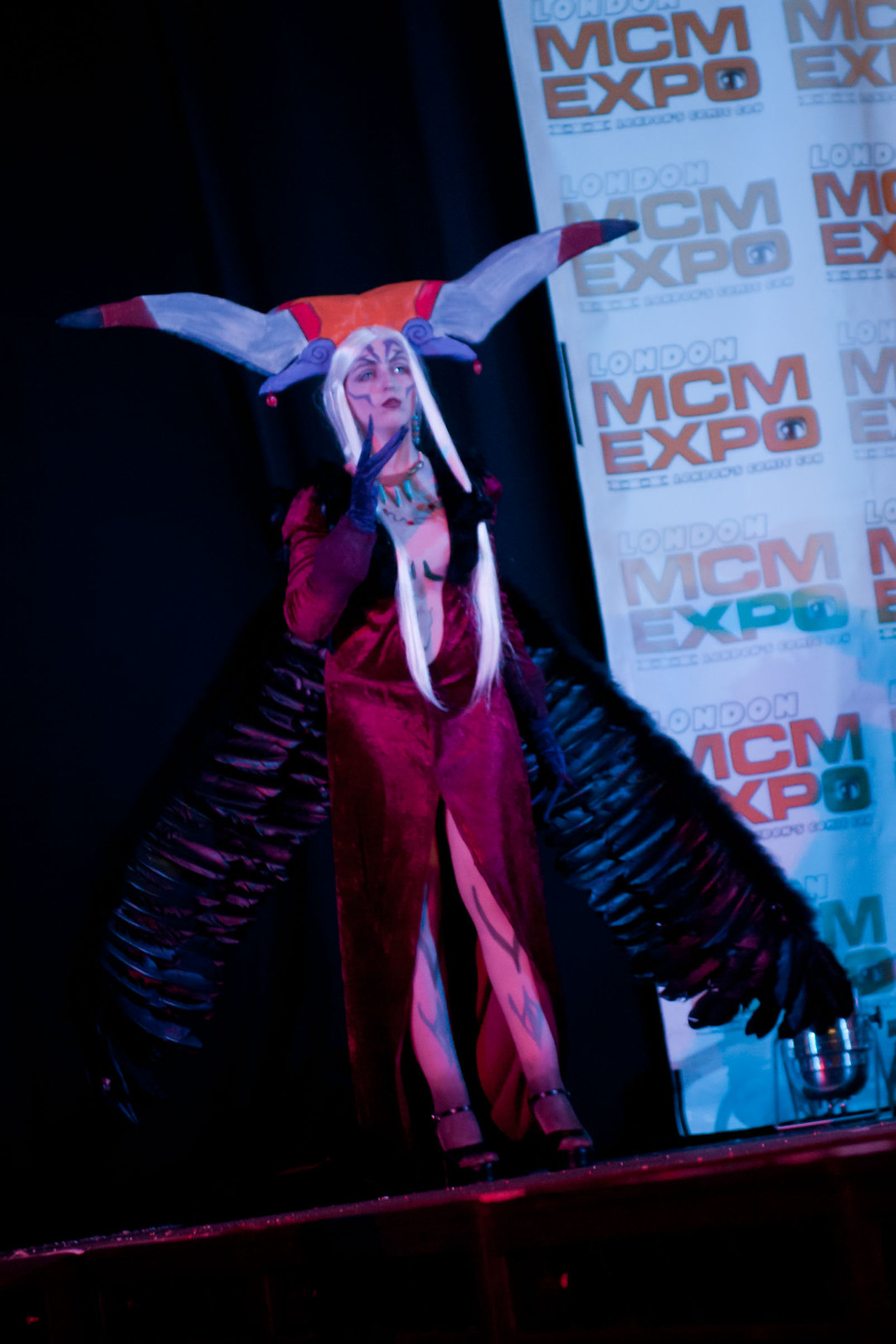In the image, a woman is standing on a stage at the London MCM Expo, as indicated by the repeated banner in the background with a white backdrop and orange text. She is dressed in an elaborate costume that features a scantily-clad red dress with an open front, revealing her chest, stomach, and legs. The outfit is accented with striking black feathered wings and large horns, which are red at the center and transition to white and black at the tips. She wears black high heels and has straps around her ankles. Her face and body are adorned with intricate paint, including black lines and stripes, and she sports red lipstick and eye makeup. Additionally, she appears to be wearing a Native American-style necklace with turquoise jewels and possibly feathered gloves. One arm is raised in front of her face, capturing the attention of the audience before her.